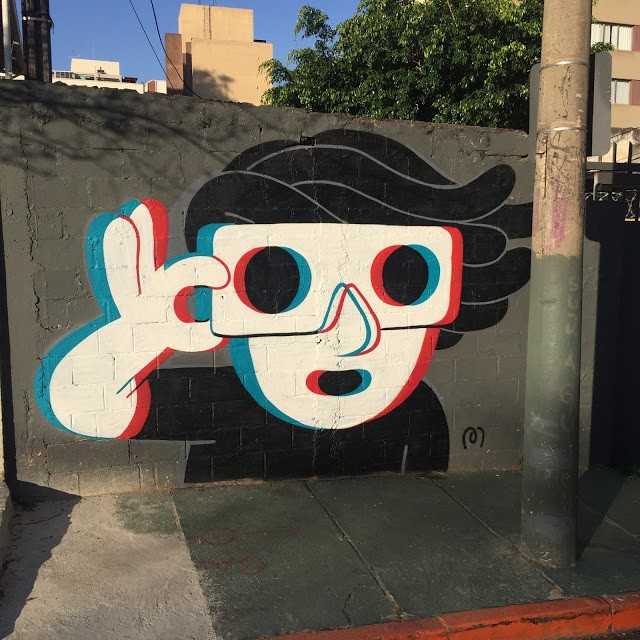The photograph captures a square mural painted on a dark gray cinder block wall along a city sidewalk. In the background, several multi-story buildings and a large green tree rise above the wall, with a blue sky overhead. The mural features a stylized image of a man with wavy black hair blowing to the right, dressed in a black short-sleeved shirt. His white face and arm are outlined with offset blue and red shadows, mimicking the effect of a 3D image viewed without 3D glasses. Ironically, the man is depicted wearing a pair of white 3D glasses that also have the red and blue outlines. To the right of the wall stands a large metal pole, similar to a streetlight, and the cement floor of the sidewalk is visible below.